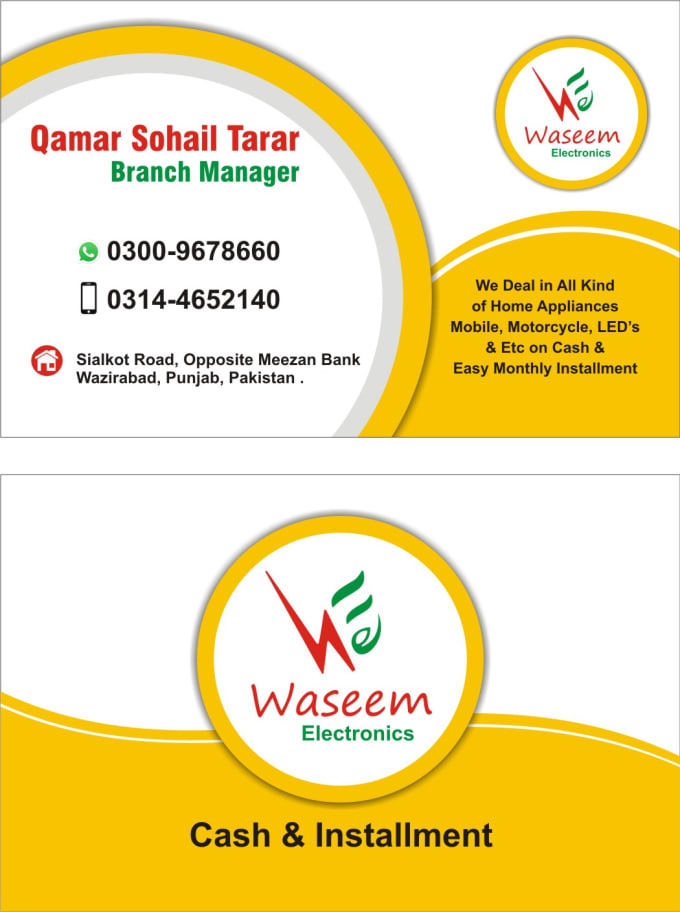This image shows a vertically oriented business card comprising both the front and back designs stacked atop each other. The upper card displays a white background with distinct sections including three yellow squares. To the left, in red text, it reads "Kamar Sohail Tarar," identifying him as the "Branch Manager" in green text. Below this, his contact information is listed: WhatsApp number 0300-967-8660 and mobile number 0314-4652-140. An address follows: "Sialkot Road, opposite Meezan Bank, Wazirabad, Punjab, Pakistan."

To the right of this section is the circular logo of "Waseem Electronics" adorned with a lightning bolt and green squiggles above the word "Waseem" which is written in red. Below this circular logo, in black text, the card states: "We deal in all kinds of home appliances, mobiles, motorcycles, LEDs, etc. on cash and easy monthly installment."

The lower card, seemingly the card's front, features vibrant yellow, green, and red colors. The logo of "Waseem Electronics" from the upper card appears again, centrally placed. The text around it highlights, "cash and installment" in black. The design incorporates a yellow swoop wave at the bottom, creating a cohesive theme for the business card.